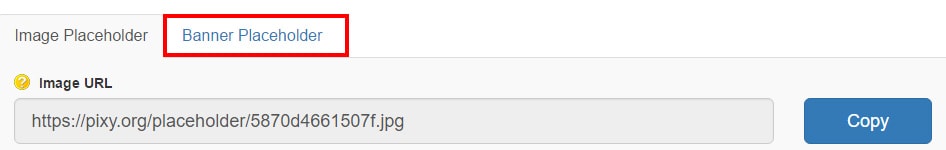Here’s a cleaned-up and detailed description:

---

The image is a screenshot of a section from the top of a website banner, although part of it is incomplete. The visible section is a narrow, gray box. This gray box has two tabs:

1. The first tab is labeled "Image Placeholder." It is active and shown in black lettering.
2. The second tab, which is not active, is labeled "Banner Placeholder." It is displayed with white text and outlined in blue lettering with a thin red box around it.

To the right of these tabs, within the same gray box, is a yellow icon containing a white question mark.

Directly below this, there is the label "Image URL" in black text. Underneath this, there is a long input box almost spanning the entire width of the gray box. Inside this box, there is a web address: "https://pixy.org/placeholder/5870D4661507F.jpg".

To the right of the web address input box, there is a royal blue button with the word "Copy" written in white letters. The rest of the content beyond this point is cut off in the image.